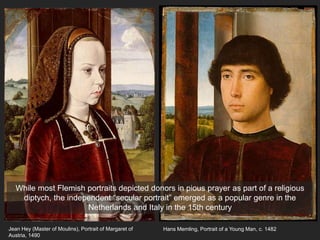This image showcases two side-by-side 15th-century portraits, exemplifying the emerging genre of independent secular portraiture in the Netherlands and Italy. Both subjects, a woman on the left and a man on the right, are dressed in red velvet garments. The woman, depicted with a serious expression, wears a long, brown headpiece resembling a towel or rug, and an ornate necklace adorned with jewels. The man has dark, possibly black or dark brown, fluffy hair and ivory-colored skin, staring forward with a solemn gaze. Both paintings highlight the transition from traditional religious donor portraits to standalone secular representations.